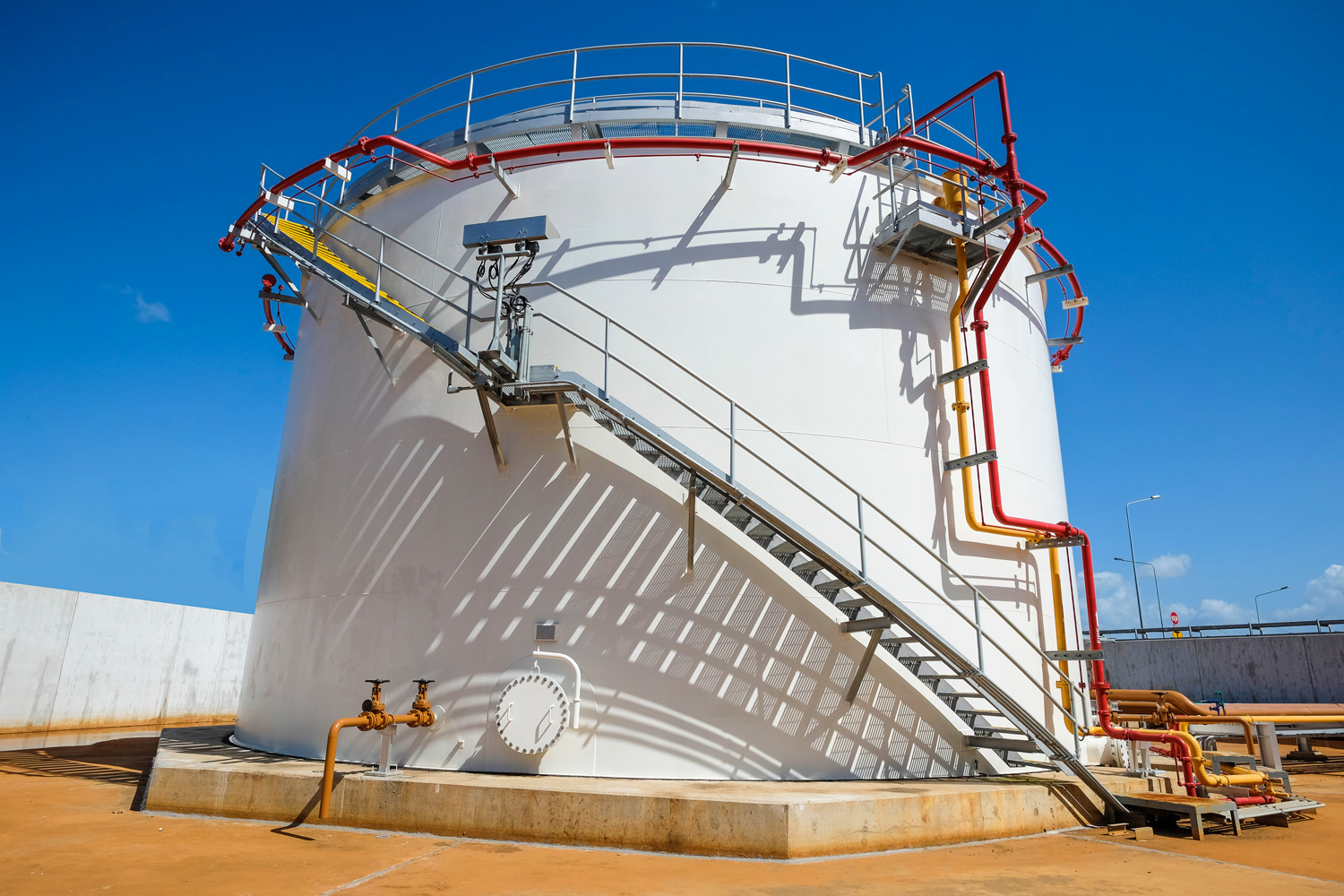This daytime outdoor photograph features a very large, round, white metal building that resembles a storage tank, possibly for water, gas, or oil. The structure stands on a square concrete base, surrounded by terra cotta tiles. A prominent gray staircase with thin handles spirals up the side of the tank, leading to a thick, rounded metal guardrail at the top. Various pipes in distinctive red and yellow colors are visible, running from the top of the tank down to the ground, with some valves apparent. In the background, a concrete divider and a stop sign can be seen, along with street lamps illuminating the area. The bright blue sky with a few clouds above completes the scene, casting a shadow of the staircase on the base of the tank, adding a striking visual effect. The entire setup gives the impression of a secure and functional industrial facility.